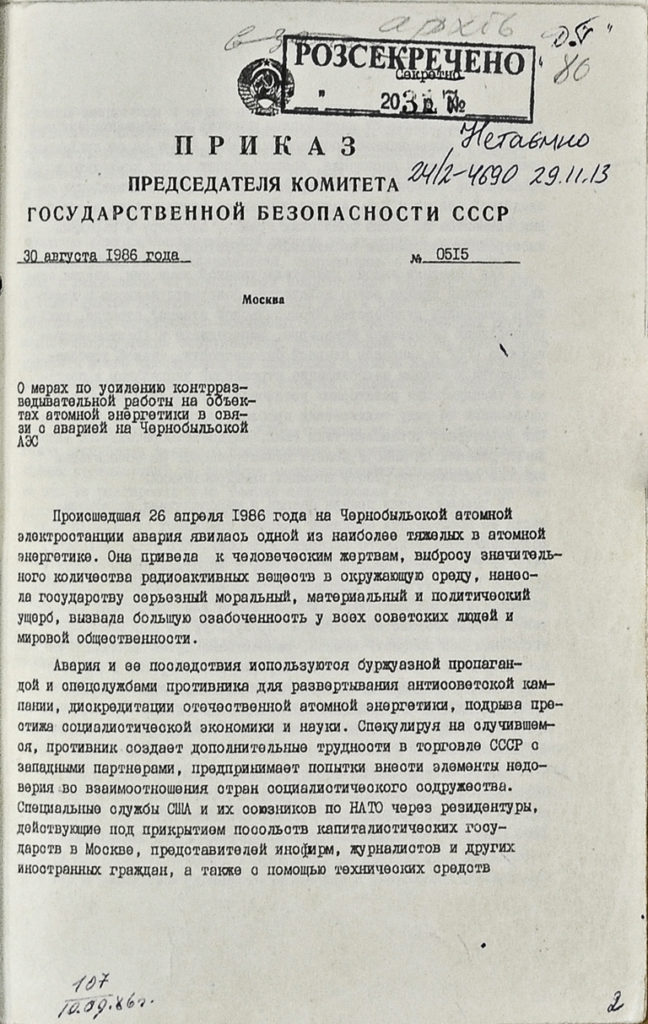This image displays an aged letter document, likely a Xerox copy, written entirely in Russian with black ink on white paper. At the top of the letter, there is a series of stamps and seals, including a rubber stamp labeled "PO3CEKPE4EHO" in capital letters. Centrally aligned below these stamps are bold headings, followed by smaller text. The date "30" and the year "1986" are clearly visible, suggesting the document is from 1986. Additionally, there's a handwritten notation in pencil and ink near the top, indicating the number "0515". Further down, handwritten markings appear again, with the number "2" inscribed in the lower right-hand corner, and another date, "26" of an unspecified month in 1986, is mentioned within the text. The document features multiple small texts, highlighting its detailed and official nature, reminiscent of the former Soviet Union era, as indicated by the appearance of "CCCP" in the third line.